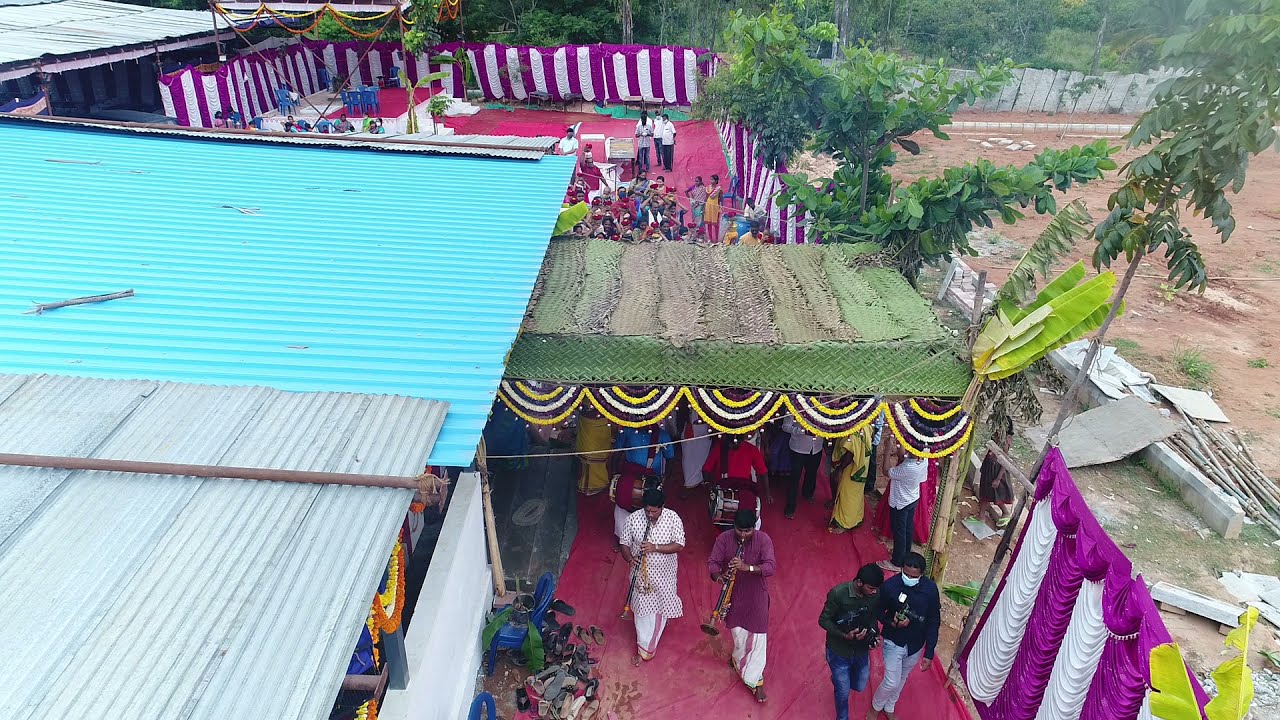The image captures an aerial view of a vibrant outdoor celebration in a village courtyard. Various buildings with colorful roofs—gray, blue, and green—enclose the festive area. The scene is teeming with people, many of whom are playing musical instruments and engaging in lively conversation. Centrally located is a green roofed walkway, beneath which stands a dense crowd, some dressed in colorful clothing, and a few men in white shirts and black pants. The far end of the courtyard features a makeshift stage, likely hosting performers.

Adorning the celebration space are walls of fabric in mixed shades of purple, white, and yellow, delicately draped to create a festive atmosphere. These fabric dividers line the area, creating semi-enclosed spaces, with some sections displaying overhead semicircle decorations of yellow and white, complete with dangling lights. A red carpet or fabric on the ground adds to the colorful decor.

In the foreground, two men—one in a white and red dotted shirt playing a wind instrument and another in a burgundy shirt with white trousers playing a black horn—entertain the attendees. Nearby, two individuals with cameras capture the ongoing festivities, while numerous shoes are neatly placed to the left, indicating an area where attendees have removed their footwear. 

To the far right, the scene transitions from vibrant activity to a barren area of brown dirt, scattered with construction materials and dotted with a few trees against the fabric wall backdrop. The left side of the image displays a building with a distinct corrugated metal roof, contributing to the rustic charm of this lively village celebration.